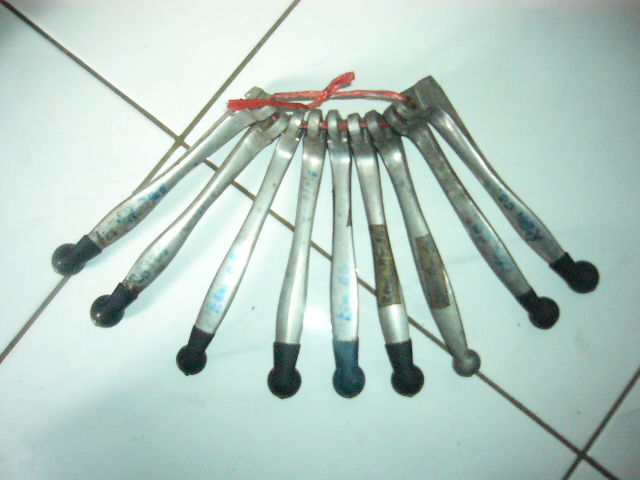This color photograph depicts nine silver metal instruments laid flat on a white tiled floor. Each instrument ends in a black rubber cap with a circular tip. The instruments are bound together at the top by a red twisty tie or string inserted through holes in the ends. Labels are present but illegible. The exact purpose of these tools is unclear; they somewhat resemble measuring spoons or reflex testers, which are typically used to tap something. The photo contains no people, animals, plants, buildings, or vehicles.